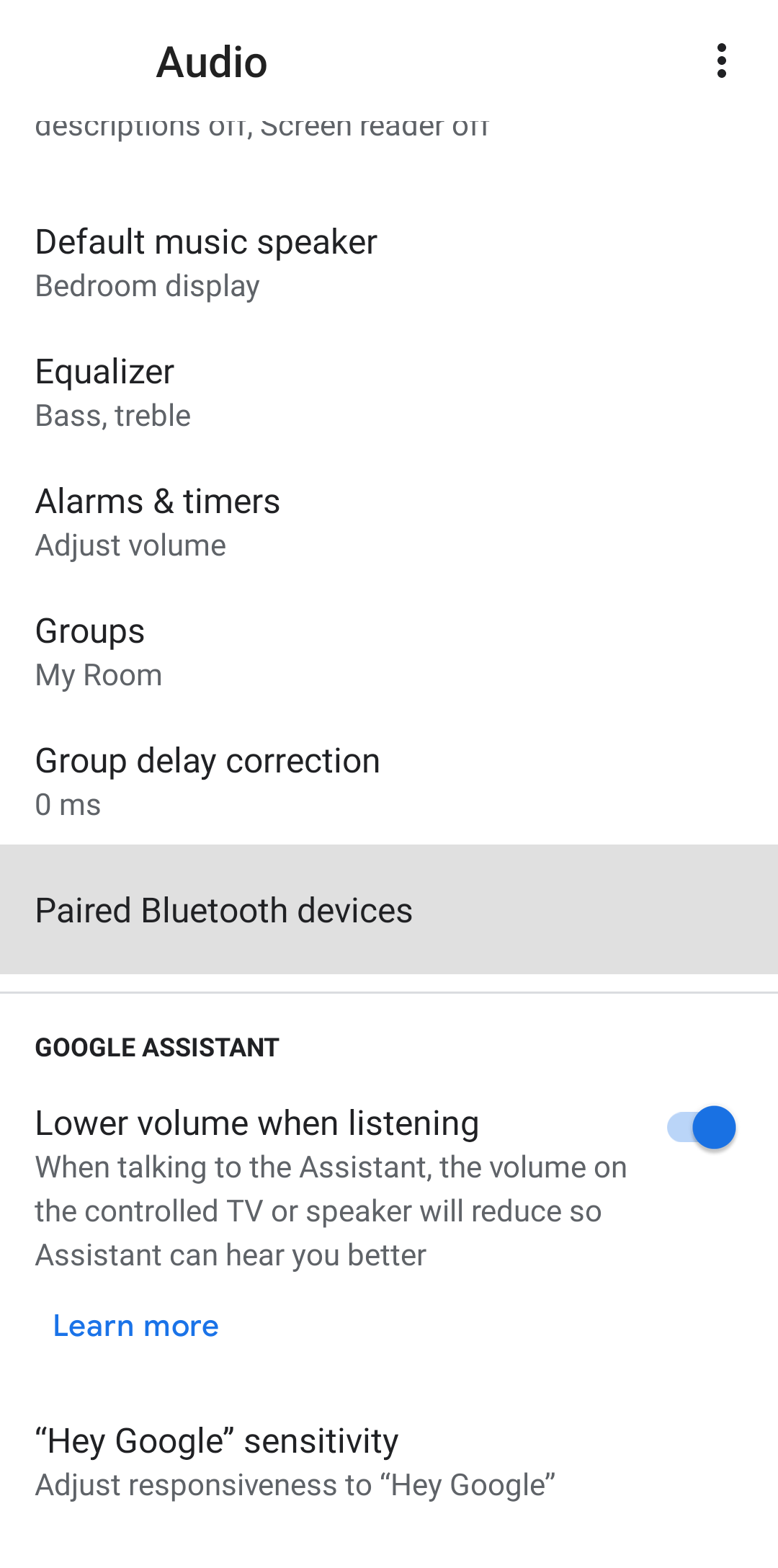This is a detailed screenshot from a mobile device displaying an audio settings page. The UI elements at the top and bottom of the device are not visible. At the very top, the page is titled "Audio," with a three-vertical-dots icon on the right, likely for accessing settings or additional options.

Below the title, there is a list of text related to audio configuration. The text, though partially cut off, is readable:

- "Descriptions off"
- "Screen reader on"

Following this, a series of subheadings with smaller explanatory text are listed:

1. **Default Music Speaker**
   - "Bedroom Display"

2. **Equalizer**
   - "Bass and Treble"

3. **Alarms and Timers**
   - "Adjust Volume"

4. **Groups**
   - "My Room"

5. **Group Delay Correction**
   - "0ms"

A highlighted heading in gray follows:

- **Pair Bluetooth Devices**
  - "Google Assistant"
  - "Lower Volume While Listening" (This option is toggled on)
  
  Under this, the description reads:
  - "When talking to the Assistant, the volume on the control TV or speaker will reduce so Assistant can hear you better."

There is a blue button labeled "Learn More" under this section.

Below, another entry reads:

- **"Hey Google" Sensitivity**
  - "Adjust responsiveness to 'Hey Google'"

The color scheme of the interface is minimalist, primarily consisting of white, gray, and black, with some blue accents. The toggle button and the "Learn More" button are blue, providing visual distinction.